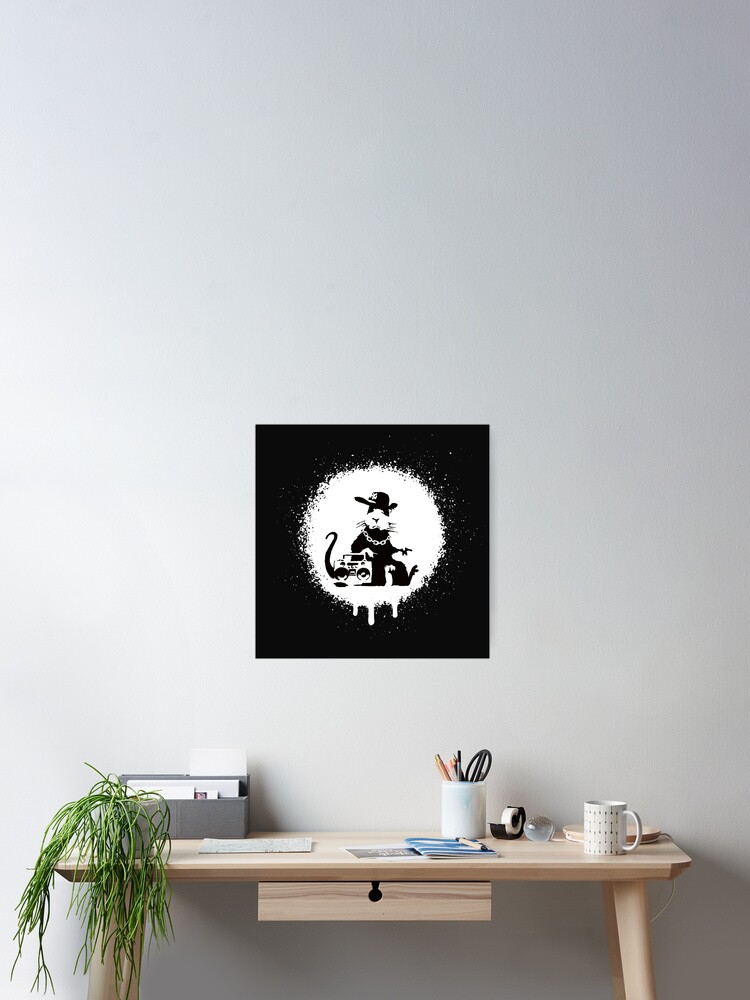In the image, a minimalist, light wood desk with slender legs and a single small drawer is positioned against a bright white background. The desk hosts a variety of items: on the left side, a verdant plant with fronds cascading over the edge from a white planter, next to which sits a gray holder containing documents. Scattered across the desk surface are a few sheets of paper, a tape dispenser, and a white mug with a pattern. A jar filled with writing utensils, including pencils and scissors, sits nearby. To the right is an extendable white lamp. Above the desk is a striking black and white picture mounted on the wall, depicting an animal in the center—possibly a cat or otter—wearing a hat and situated within a white circle that appears to be dripping slightly, all set against a black background. The overall aesthetic is simple and artistically inclined, with emphasis on light tones and functional yet elegant decor.